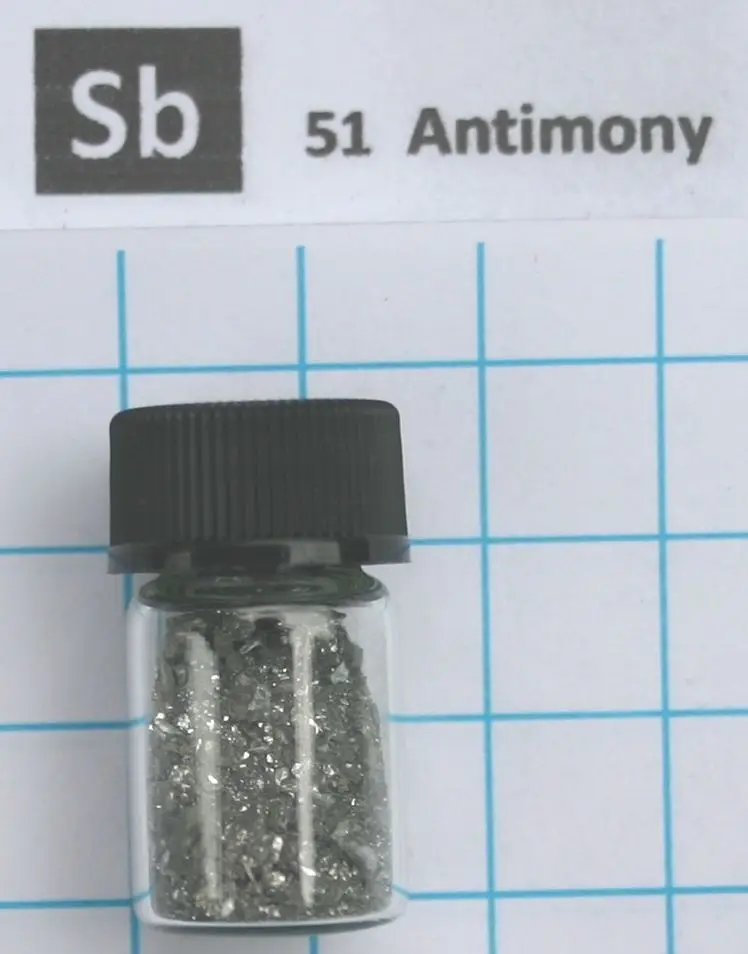This photograph features a small clear glass bottle containing pieces of Antimony, a silvery-white metal, with some pieces appearing shiny and others more matte gray. The bottle, which has a large black twisty cap, is resting on a paper with a blue and white checkered graph pattern, likely for measuring the height of its contents. Positioned above the bottle, a black square displays "SB" in bold white print, followed by the number "51" to its right. Further to the right, the word "Antimony" is printed prominently in black on a white background, with "Antimony" in capitalized and the surrounding text in smaller letters.